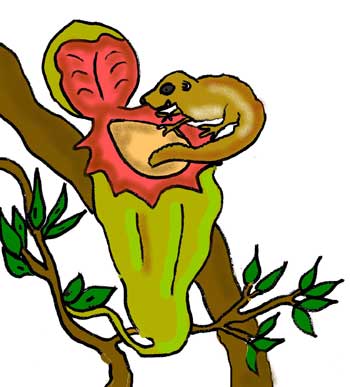This cartoon image features a detailed scene set against a white background. At the center of the image, a small brown squirrel with a curled tail and a prominent black eye is perched on the red edge of a large, green, acorn-shaped fruit. The fruit, which has an acorn-like shape with a green exterior and red edges, sits on a branch that extends from the lower right diagonally to the upper left. The lid of the fruit is lifted, revealing a pink inside with a green top on the lid.

The branch holding the fruit is supported between two larger branches, with an array of green leaves scattered around. Leaves extend towards the right side and the upper left, contributing to the natural, outdoor setting of the drawing. In addition to the squirrel, a green lizard can be seen on the red border of the fruit, adding more life to the scene. The combination of light green, light red, tan, brown, and dark green colors enhances the playful and detailed nature of this artistic depiction of wildlife.